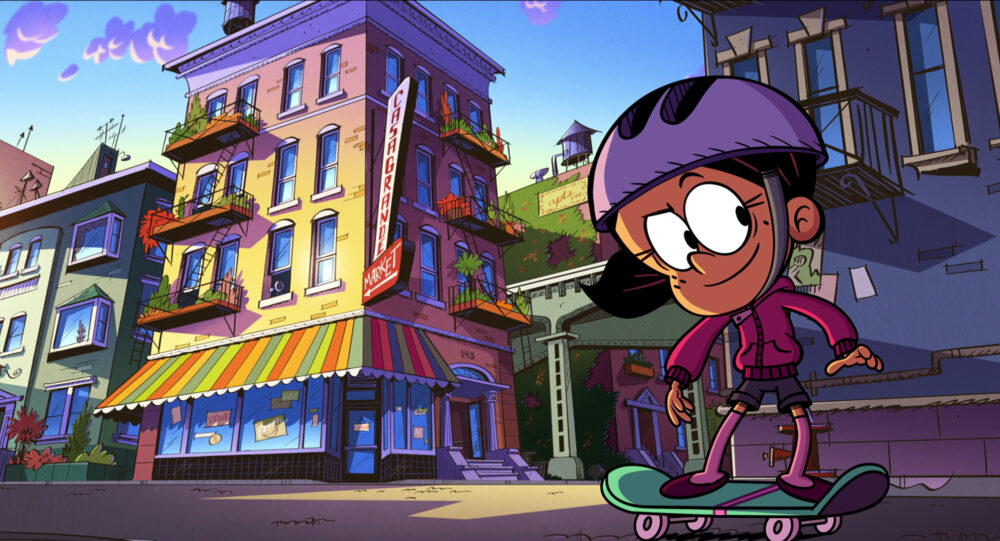In this vibrant scene from the cartoon "The Casagrandes," produced by Cartoon Empire, a young girl, approximately four or five years old, is energetically skateboarding down a concrete sidewalk. She sports a pink jacket, pink or purple shorts, contrasting long pink or purple socks, and vibrant purple shoes. Her dark brown hair is protected by a purple helmet, and she rides a mint green skateboard adorned with pink wheels and a pink stripe. Her large, white eyes reflect her lively spirit as she passes by a bustling downtown area.

The backdrop predominantly features a three-story building with an eye-catching, multi-colored awning that includes hues of red, blue, green, and white, wrapping around the glass-fronted market below, labeled "Casagrande Market." This market, adorned with rainbow-colored details and surrounded by street-level ads, gives way to the residential upper floors with balconies festooned with green and red plants. Adjacent to this, a greenish building and a neighboring blue brick structure hint at more residential spaces above the street-level shops. The scene perfectly encapsulates the lively, colorful essence of the show's urban setting.